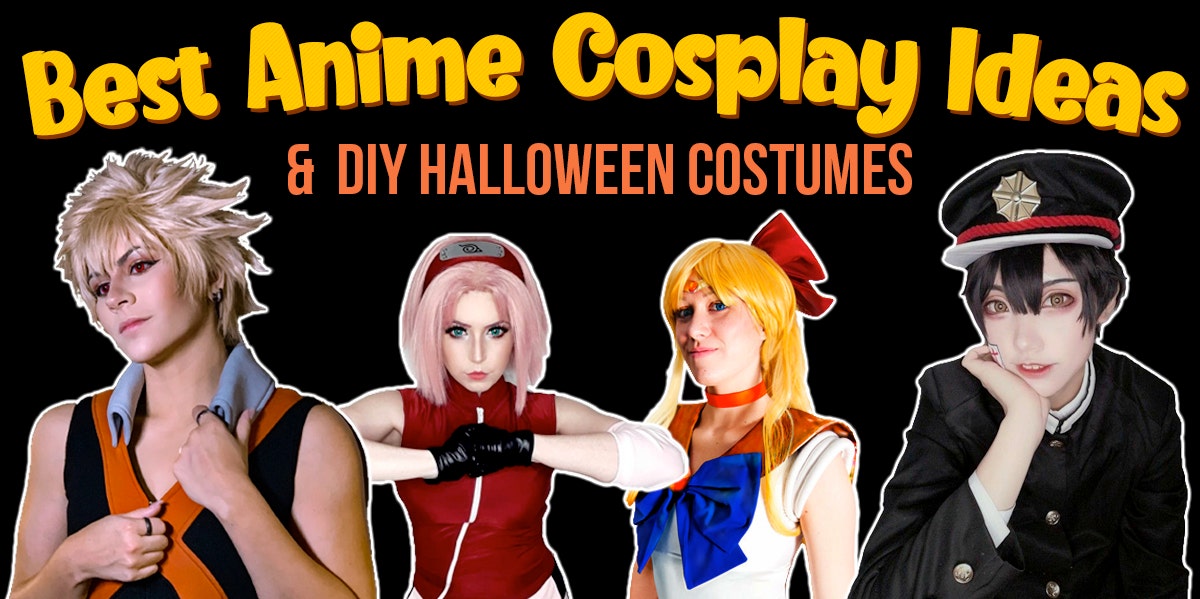The image has a YouTube thumbnail style, featuring a solid black background with text at the top. The top caption, in yellow bubbly font, reads "Best Anime Cosplay Ideas," while a bold, light orange text underneath announces, "DIY Halloween Costumes."

The image displays four individuals in elaborate cosplay outfits:
1. The leftmost character cosplays as Bakugou from *My Hero Academia*, distinguished by white, spiky hair and an orange and black top.
2. Next to them is a cosplayer in a red outfit with pink hair, likely inspired by a character from *Naruto*.
3. The third character is dressed as Sailor Moon, wearing her iconic outfit with yellow hair, a large red bow, a blue bow on her top, and a gold collar.
4. The far-right cosplayer is dressed in a black outfit, featuring a black hat with a red band or rope surrounding the brim and gazing directly at the viewer.

Each cosplayer is meticulously styled, showcasing their dedication to recreating these famous anime characters, perfect for offering unique ideas for anime cosplay or DIY Halloween costumes.